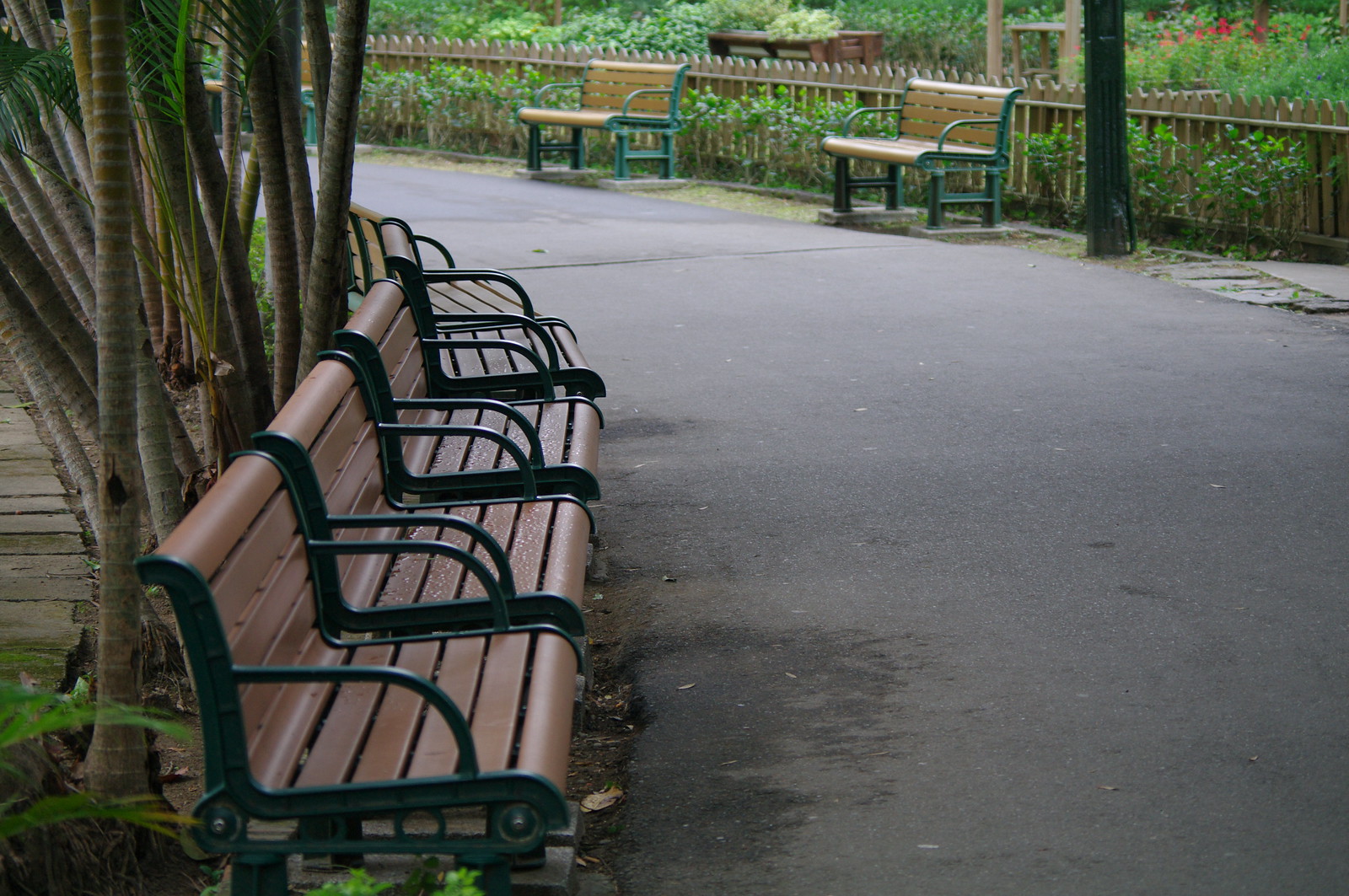This photograph captures a park featuring a wide, paved trail that circles around the entire area. The trail starts from the bottom right corner of the frame, extending to the upper left, becoming narrower in the distance as it curves to the left. Surrounding the outer edge of the park is a four-foot-high wooden fence intertwined with green leaves, giving it a harmonious, natural look.

Adjacent to this trail, numerous wooden benches with green metal frames are placed at regular intervals of about ten feet. These benches have medium-colored wooden slats and appear to have handles, which are particularly visible on the benches closer to the camera, showing a morning dew on their surface. In the park's center, there is another set of similar benches arranged much closer together and curving around a stand of thin, tropical-looking trees, which likely belong to the southern hemisphere. Beyond these inner benches, a wooden walkway can be seen extending into the greenery.

The park is lush with green plants and shrubs, providing a serene and natural atmosphere. Amongst the greenery on the right side of the image are more benches, consistent in design with green metal arms and legs, contrasted by tan-colored wooden seats and backings. Behind these benches is a continuation of the brown picket fence. Overall, this detailed view highlights the park's blend of structured pathways, comfortable seating, and rich vegetation, making it an inviting space for visitors.